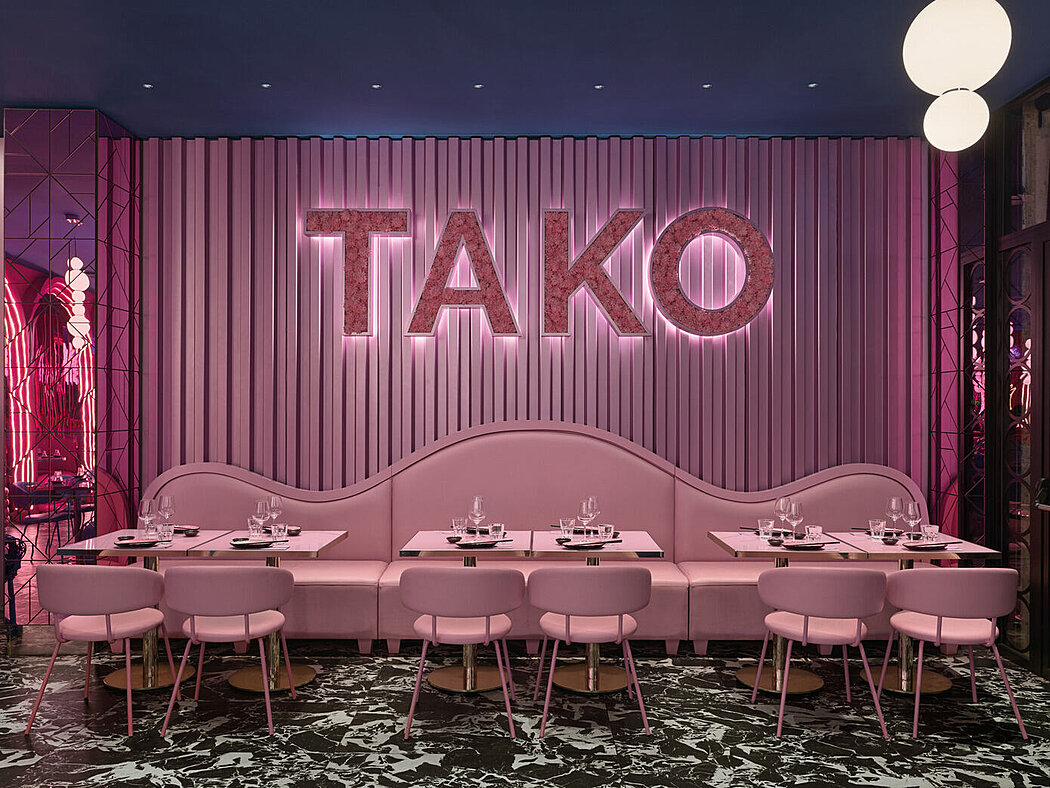The image is a detailed 3D color illustration of a restaurant or lounge interior, likely created in an app like SketchUp. The setting is a landscape-oriented room with a distinctive ambiance. Its ceiling, dark and blackish, features small overhead lights casting a soft glow. Along the back wall is a prominent purplish curtain, vertically striped and adorned with the word "TAKO" spelled out in three-dimensional, backlit chrome letters.

The seating arrangement includes a vibrant pink banquette sofa that spans horizontally across the bottom third of the image, curving slightly higher in the center. In front of the banquette, there are three sets of tables, each formed by two smaller tables pushed together, making a total of six. These tables are adorned with clear glass place settings, including wine glasses, small water glasses, plates, and small dishes that suggest a spicy condiment.

Facing the banquette are six pink chairs with metal legs, two at each table. The tables themselves have pedestal bases and round brown bottoms, with rectangular pink tops. To the left, a lit decorative feature that resembles a round archway adds to the room's stylish decor. Reflective mirrored panels are present on both the right and left sides of the space.

Above, the ceiling bears distinctive small overhead lights, with a notable light fixture on the top right consisting of two white balls, a larger one above and a smaller one below. Completing the setup is a dark green carpet with a white abstract pattern, indicative of a chic, modern aesthetic.